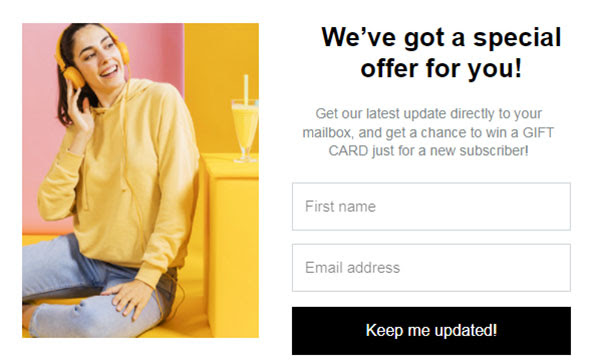The image displays a vibrant promotional pop-up ad with a special offer encouraging user engagement. Dominating the visual on the left is a stock photo featuring a young woman clad in yellow attire – a yellow over-the-ear wired headphone set, yellow hoodie, and light blue jeans. She stands against a predominantly yellow room, complete with a yellow smoothie in a glass, which contrasts with a segment of a pink wall, creating a lively and colorful backdrop.

On the right side of the ad, the promotional text invites users to receive the latest updates directly to their mailbox and enter for a chance to win a gift card by subscribing. To participate, users are prompted to enter their first name and email address. Below the input fields, there is a prominent black button with white text reading "Keep Me Updated." This ad subtly conveys an enticing offer amidst a visually engaging scene dominated by cheerful yellow tones, aimed at attracting potential subscribers.